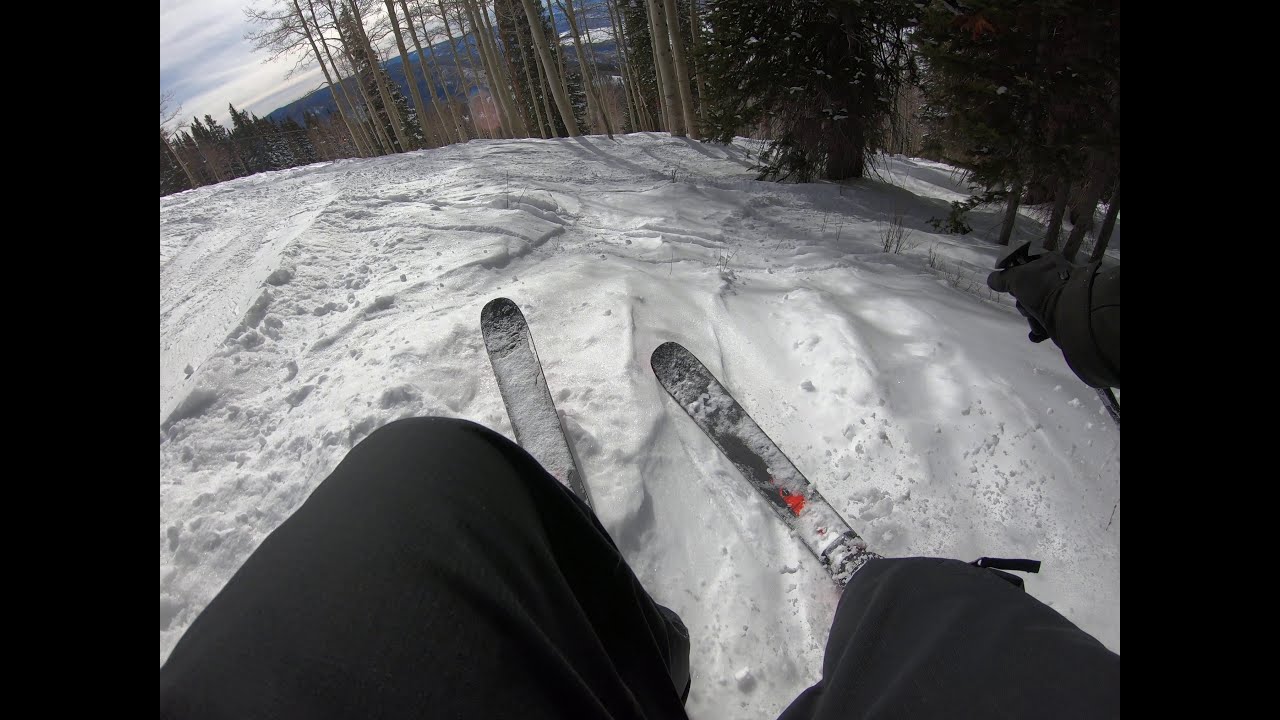In this detailed landscape-oriented, color photograph, a skier captures a dynamic point-of-view shot as they descend a snowy hillside. The skier's black skis and part of their black-clad knees are visible at the bottom of the frame, aimed slightly towards the upper left corner. Snow is kicked up around the skis, emphasizing the action of the descent. 

The scene is dominated by a snowy ground dotted with various trees, including bare and pine varieties. To the right, a dense section of dark woods and dead trees edges the snow-covered slope. The upper left of the image features an enormous, heavily clouded sky that stretches above a faint, hazy mountain range in the distance. A bright patch of snow stands out behind one of the trees, contrasting with the overall grey and white tones of the landscape. The photograph, a freeze-frame from a GoPro video, exhibits a style of photographic representationalism, capturing the raw realism of the skiing experience.